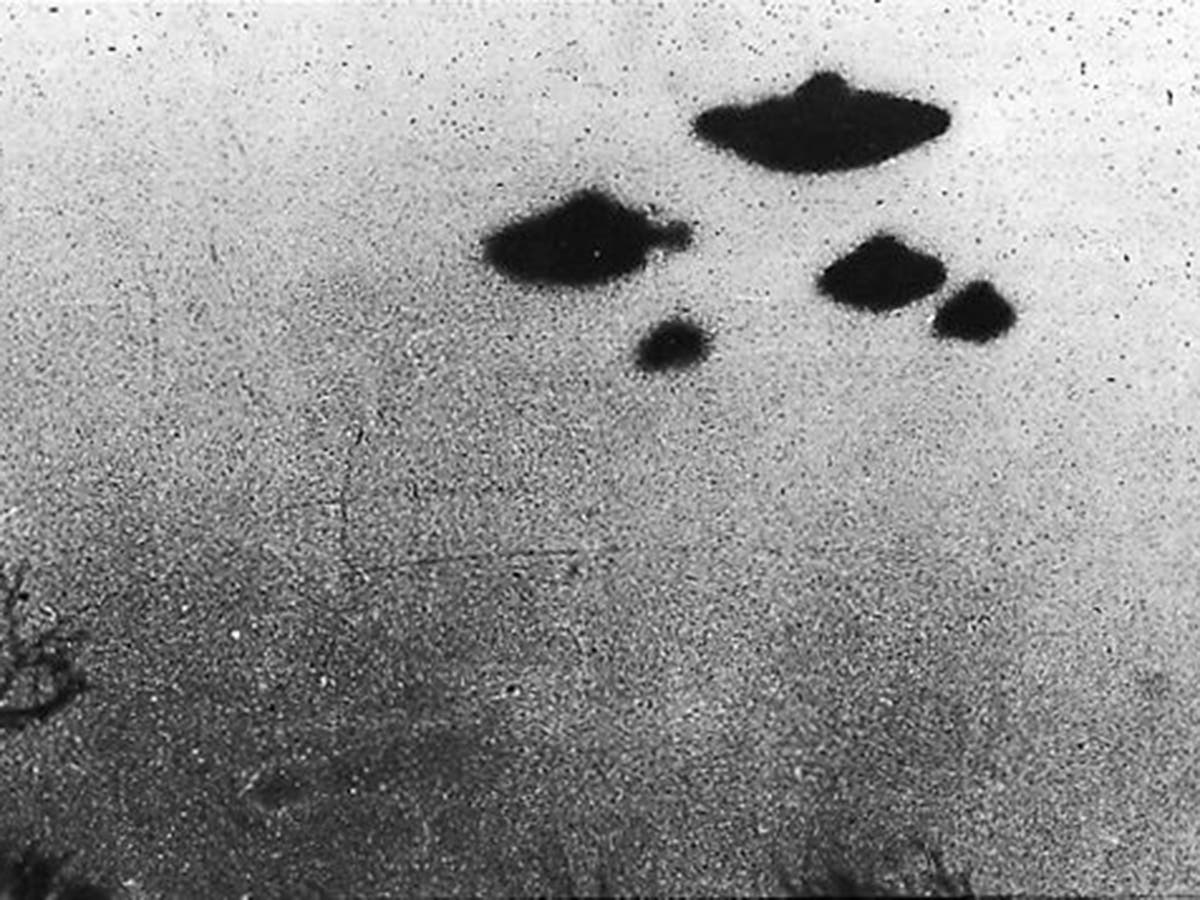The black and white photo, though heavily distorted and grainy, captures five shadowy objects in the sky, positioned in the top right corner. Among these, one object resembles a classic flying saucer with a disc-like shape and a dome-like center. The other objects share a similar saucer-like appearance but vary in size, suggesting differences in distance. Despite the pixelation and lack of clarity, the image clearly depicts these unidentified flying objects, which could also be misinterpreted as fish swimming underwater due to the blurriness. The photo contains no text, numbers, or letters, relying solely on the visual portrayal of these enigmatic shapes.